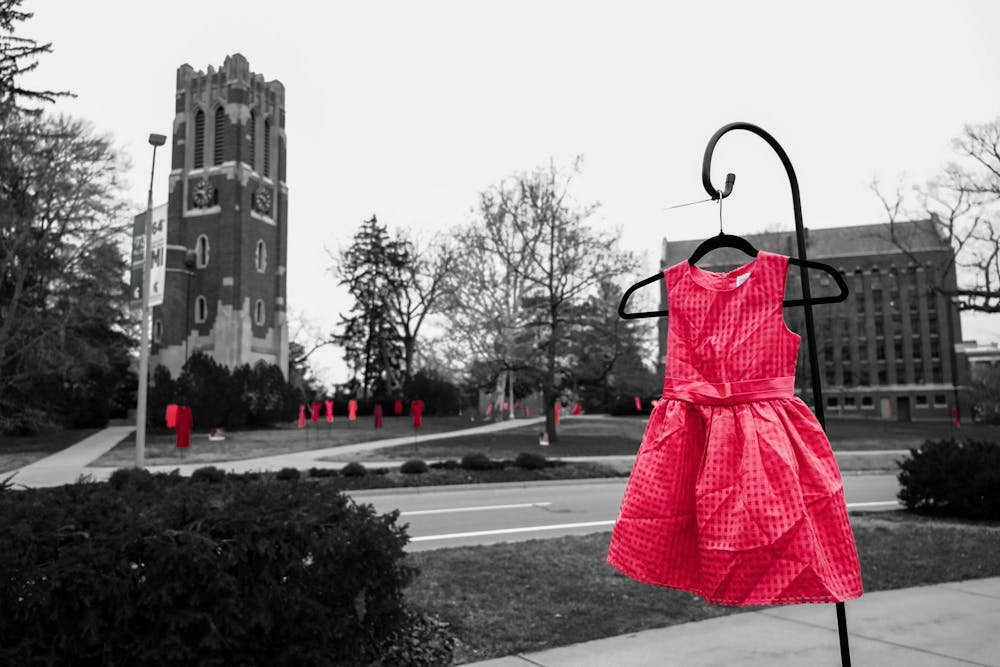This modern black-and-white photograph captures a captivating street scene dominated by an imposing building in the background, which appears to be a cathedral or church, marked by tall brick structures and a clock tower. To the right, there's another prominent five-story building, partially obscured by trees and shrubbery. The foreground of the image is strikingly contrasted by a vivid red dress, likely a pinafore, hanging from a wrought iron hook on the sidewalk, akin to a plant hanger sprouting from the ground. This dress stands out as the only splash of color, reminiscent of scenes from "The Red Balloon." Additionally, there is a series of similar red garments or flags in the background, lined up against the monochrome architecture, suggesting a symbolic significance. The scene is bordered by sidewalks and vegetation, creating a blend of natural and urban elements in a visually arresting composition.